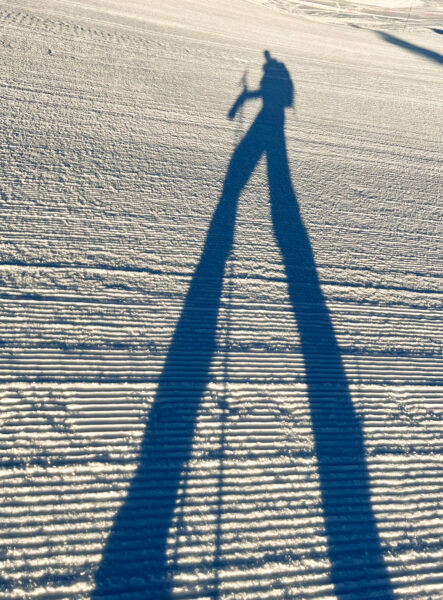The image depicts a bright, sunny day on a freshly groomed ski slope, where the low angle of the sun casts a strikingly elongated shadow of a skier. The shadow reveals the skier's body, long legs, and two ski poles, creating an almost surreal effect that makes the figure appear to be on stilts. The terrain showcases precisely graded, textured lines running across the slope, which is covered in light-colored snow. The skier's silhouette also hints at a backpack, adding to the impression of a hiker-like figure. The overall scene combines the stark contrast of the shadow with the serene, well-maintained snowy landscape, illuminated by the early morning or late afternoon sun.